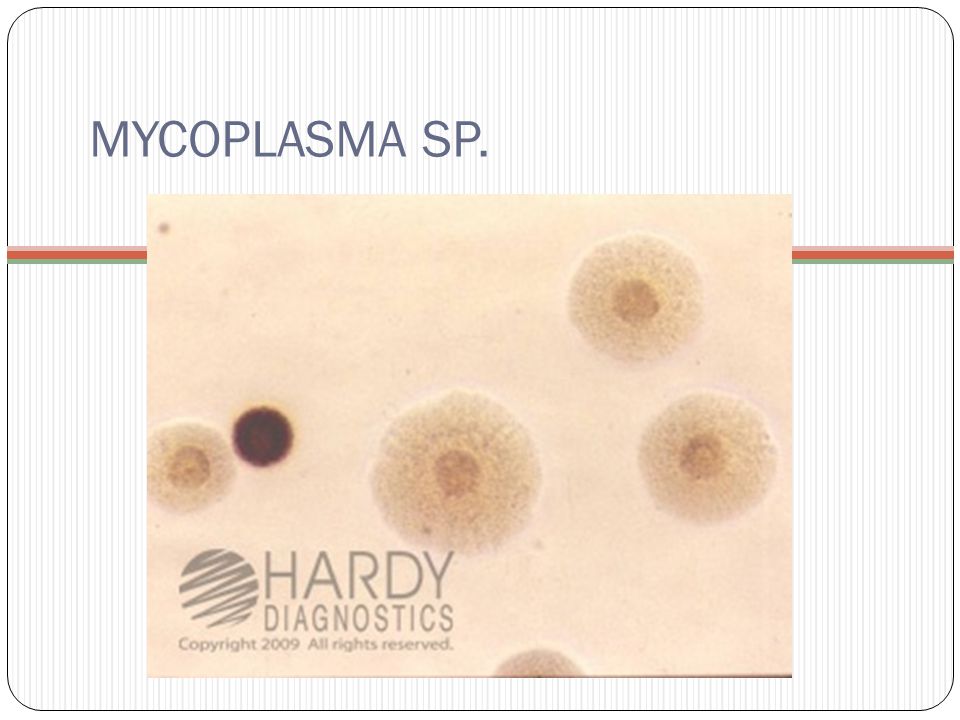The image is a digital, landscape-oriented graphic that resembles a business card or a slide from a presentation. The entire image is bordered by a thin black line with rounded corners. The background features light gray vertical stripes that provide a subtle texture. Near the top left corner, in all caps and gray font, is the label "MYCOPLASMA SP." Just below this text, there are three horizontal stripes in light pink, red, and green from top to bottom.

At the center of the image, there is a photo of Mycoplasma cells with a cream-colored background. The cells are depicted as circular, light brown structures with darker brown centers. 

In the bottom left corner of the cell photograph, there's a circular logo made up of brown scribbles. Adjacent to the logo, in all caps gray letters, it reads "HARDY DIAGNOSTICS." Below this, in smaller print, it states "Copyright 2009. All Rights Reserved."